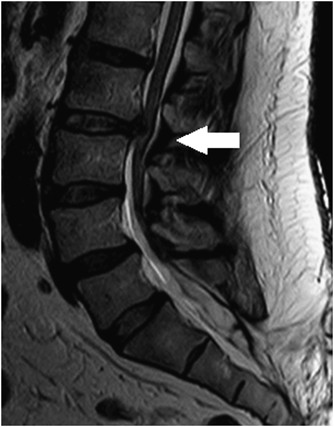This is a black-and-white, vertical portrait image, likely a medical scan such as an MRI, featuring a detailed grayscale representation of an anatomical part. A prominent white arrow in the upper right quadrant points towards the center of the image. Central to the composition is a ribbon-like structure that curves from the middle top, swooping downwards towards the bottom right corner. This structure is a gray band with a distinctive white stripe running through it. To its right is a larger, fissured gray band, approximately five times wider, stretching diagonally from the bottom right to the top right corner. Adjacent to these bands, the right edge includes a darker section resembling an esophagus-like shape. Below and to the left of these elements is a black space following the contours of the gray bands, filled with gray matter in the bottom left, forming a triangular pocket. The entire image is grayscale, showing varying shades from black to white, and includes dotted white lines in the upper right corner, simulating intricate details possibly of the internal body.